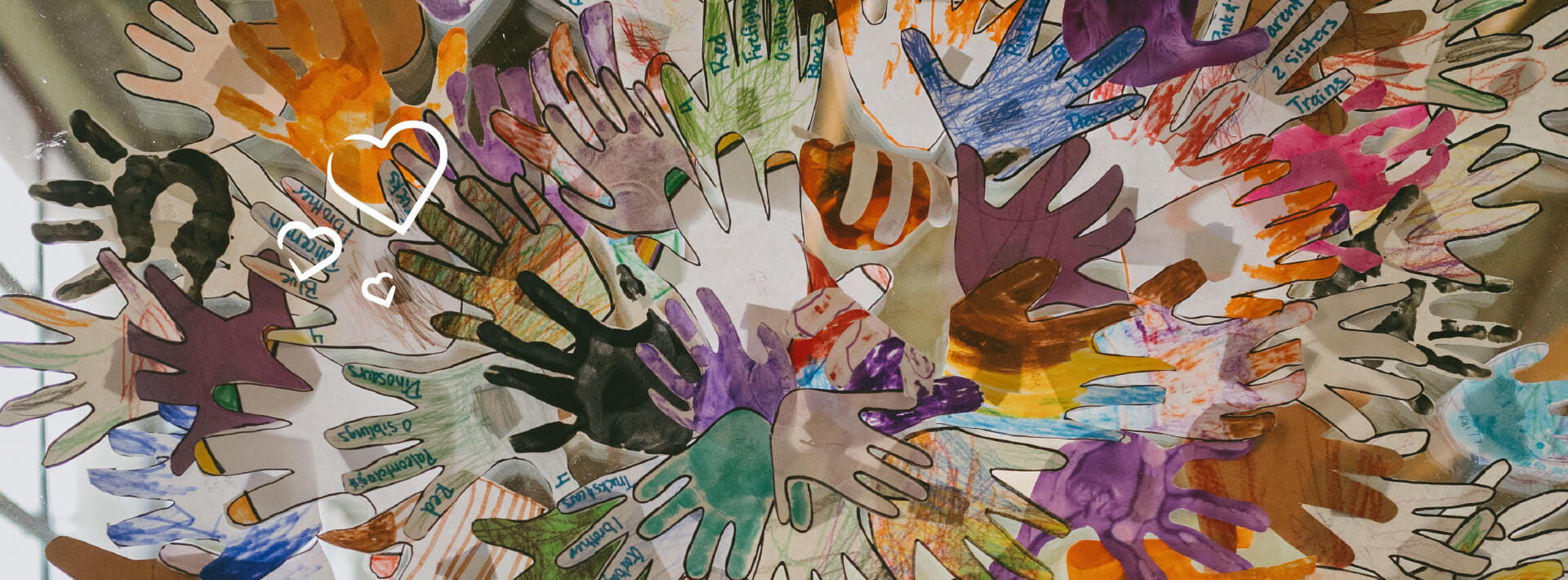The artwork is a vibrant and intricate painting that portrays a multitude of handprints, meticulously arranged to form a strikingly elaborate circular pattern. This visually engaging piece features a range of handprints that emanate from the center and spread outwards toward the edges, creating an almost floral configuration. The hands, depicted in an array of colors including white, beige, brown, gray, black, blue, purple, green, pink, and orange, are both outlined in black and filled in with a variety of hues, adding to the dynamic and textured appearance. Some hands appear to have been colored in using crayon-like strokes, enhancing the playful and diverse aesthetic. Positioned on what seems to be a glass window, the artwork allows glimpses into a blurred background that suggests a classroom setting, blending the vibrant handprints with a sense of everyday reality. This detailed and lively collage-like creation captures a rich tapestry of human imprints, symbolizing unity and diversity through its array of color and form.